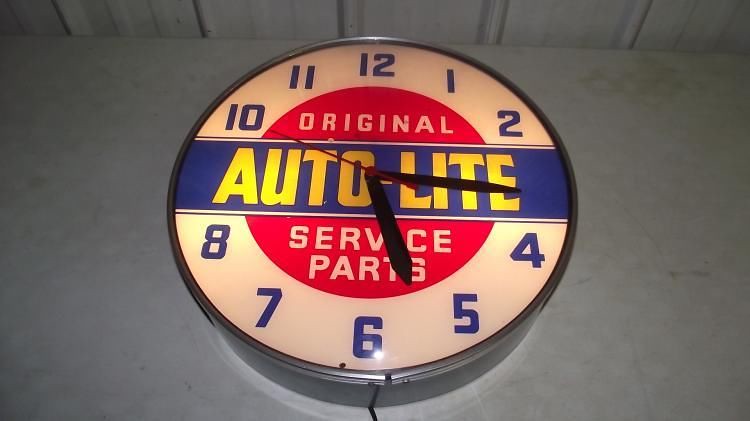The photograph captures a vintage advertising wall clock in vivid detail, showcasing excellent color, lighting, and focus. The clock, mounted high on a white wall near a metallic ceiling, is encased in a chrome frame with a slightly domed glass lens. The clock face features a white background with blue numbers, though the 3 and 9 are obscured by a horizontal blue banner. The banner bears the bold yellow text, "Autolite Original Service Parts," and intersects a solid red circle with the white words "Original Service" above and "Parts" below. The clock is illuminated, highlighting its details, and includes two black hands indicating approximately 5:16 and a red second hand currently pointing towards the 10. An electrical cord is visible, protruding from the bottom, confirming it is not battery-operated. The photograph is taken from a slightly low angle, adding a unique perspective to the scene.